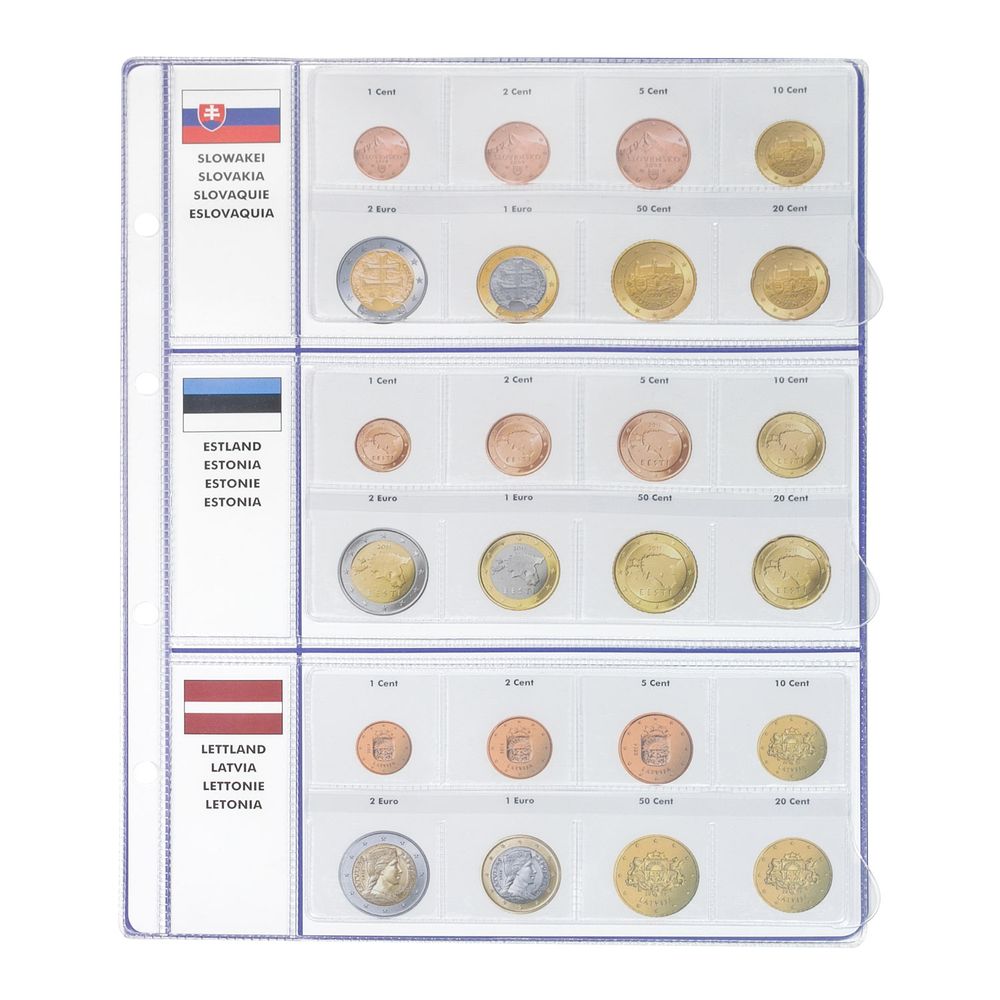The image is a detailed, brightly lit, color display of Euro coins from Slovakia, Estonia, and Latvia, divided into three sections. Each section showcases eight coins from the respective country, with their flags and country names clearly labeled. The first section, displaying coins from Slovakia, features a red, white, and blue flag and the label "Eslovakia." The middle section contains coins from Estonia with a blue, black, and white flag, labeled "Estonia." The third section presents coins from Latvia, accompanied by a red and white flag and labeled "Latvia." The coins, which mostly appear in shades of gold and copper, are neatly arranged in individual spaces, resembling the layout of a collector's album or a reference guide, with four coins in the top row and four in the bottom row of each section. The clarity of the image allows for easy visibility of the details on each coin and their respective labels, making it a precise and well-organized visual display of Euro coins from these three countries.